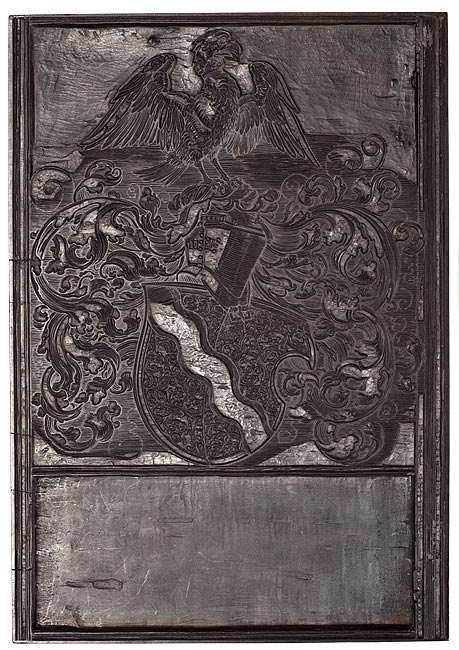The image appears to be an engraving or lithograph, possibly made from metal or wood, characterized by its dark and intricate details. The central theme of the composition includes meticulously etched designs of scrolling plants and flowers that create an almost paisley pattern. Amidst these elaborate motifs, there are two birds, potentially vultures or eagles, positioned at the top of the image. They are perched in such a way that they seem to be gazing towards the left side. Below them, a knight's helmet and shield, adorned with a wavy stripe and possibly representing heraldry, add to the ornate nature of the depiction. The knight's helmet is solid and hides the knight's face, topped with a crown that might symbolize rank or nobility. The surrounding frame is wide, with the lower portion of the panel showing some wear and tear but remains uncarved. Despite the overall dark and possibly aged appearance, the artwork showcases a high level of craftsmanship, indicating that it was a labor-intensive piece.